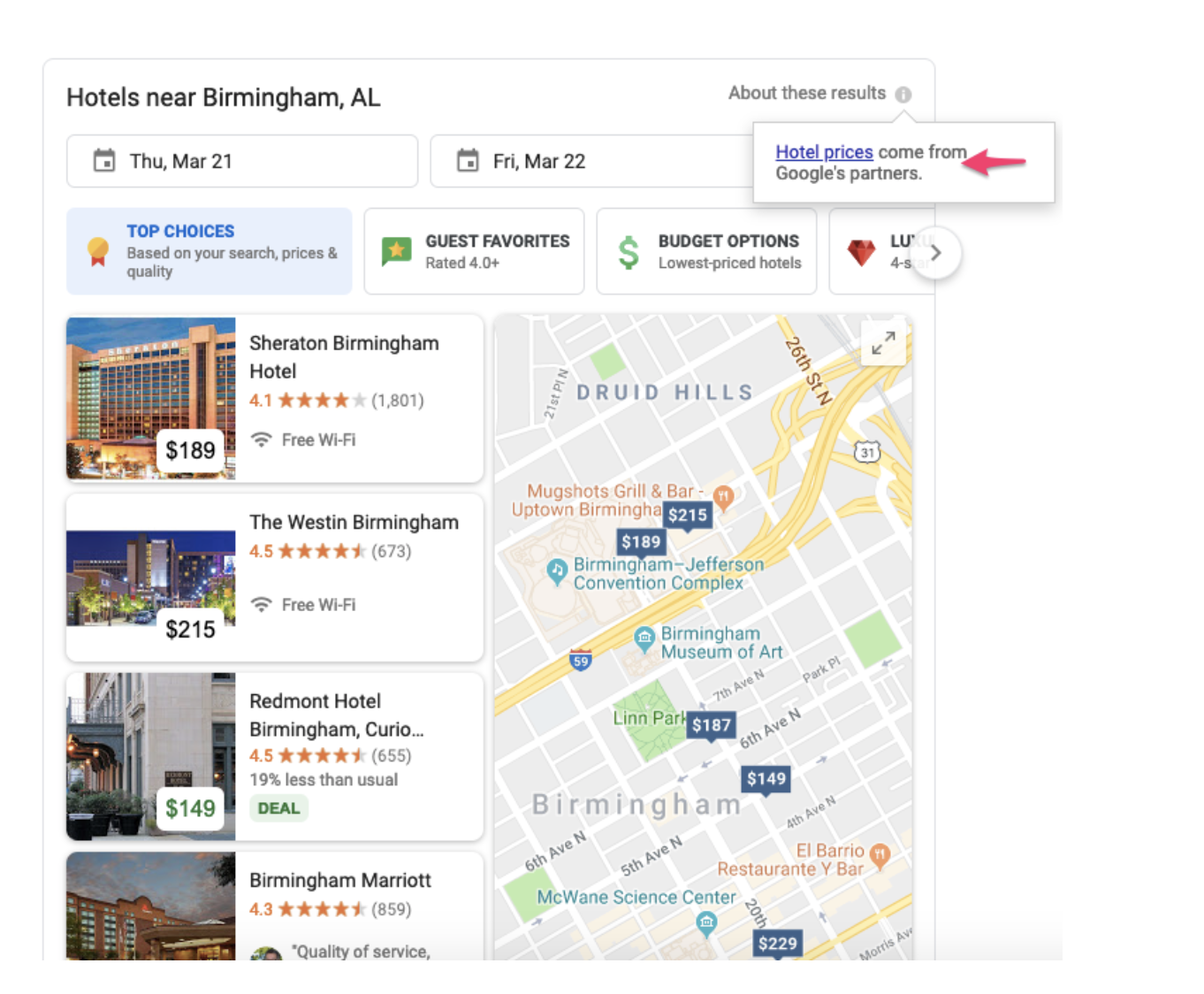This image depicts a detailed web page of a hotel search for accommodations near Birmingham, Alabama. At the top of the page, it prominently displays "Hotels near Birmingham, Alabama" followed by an option labeled "About these results." A calendar icon indicates the check-in date of Thursday, March 21st, and the check-out date of Friday, March 22nd. A note on the side mentions that hotel prices are sourced from Google's partners, with a clickable blue link marked by a red arrow. This information is displayed in standard black and white text.

Below this section, there is a header titled "Top Choices" in blue text. This area has a light blue background and includes a message in black text, "Based on your search, prices, and quality," accompanied by a gold award symbol with a red ribbon. Further down, the page categorizes hotels into "Guest Favorites," "Rated 4.0+," "Budget Options," "Lowest Priced Options," and "Luxury."

Featured hotels include:
- **Sheraton Birmingham Hotel:** Offering free Wi-Fi at $189 per night, with 1,801 four-star reviews.
- **The Westin Birmingham:** Also providing free Wi-Fi at $215 per night, boasting an average rating of 4.5 stars from 673 reviews.
- **Redmont Hotel Birmingham - Curio Collection by Hilton:** Priced at $140 per night, 19% less than usual, featuring 4.5 stars from 655 reviews.
- **Birmingham Marriott:** With an average rating of 4.3 stars from 859 reviews, stressing its quality of service.

Each hotel listing includes a photo of the property. On the right-hand side of the page, a map displays the location of these hotels and nearby attractions.